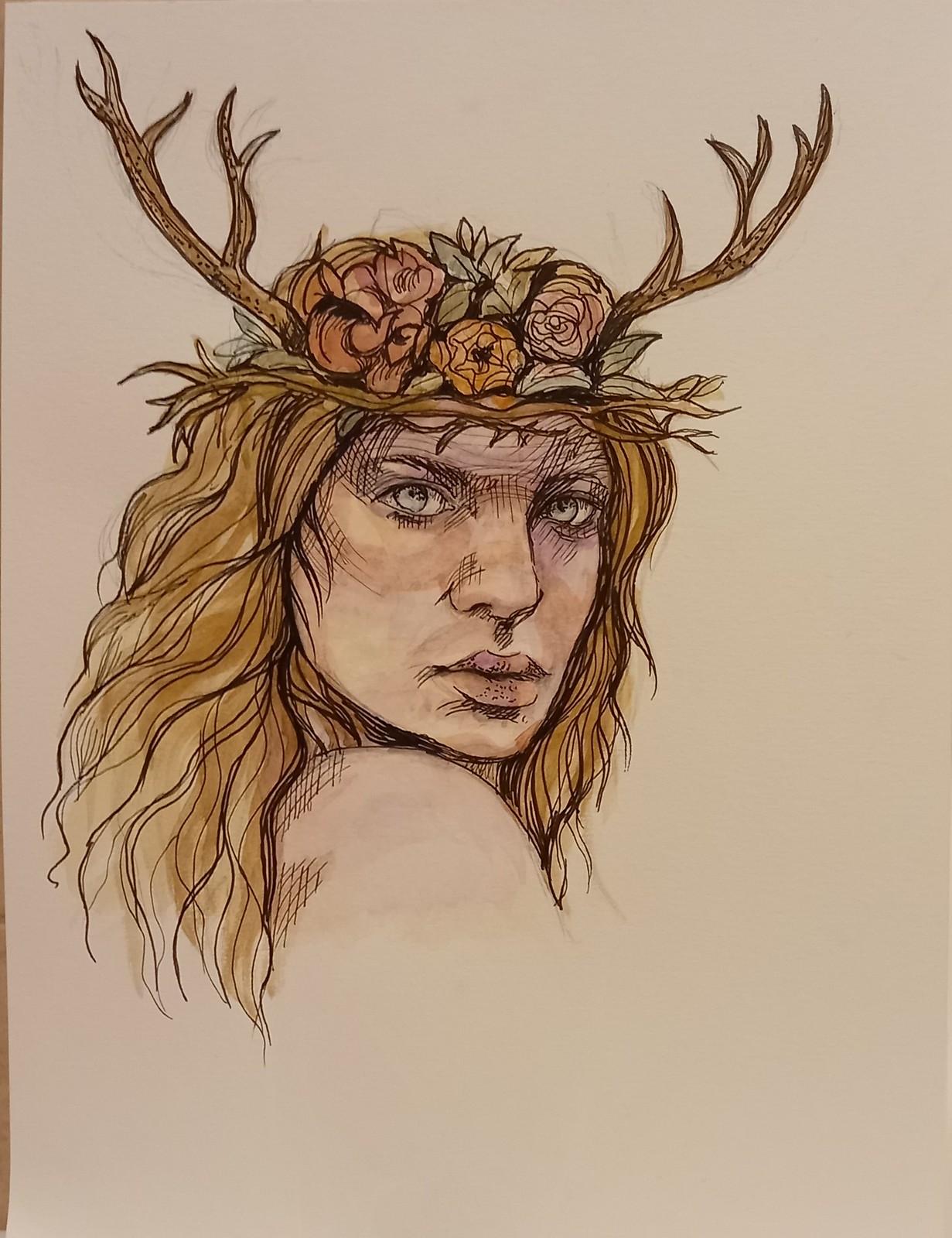This is a detailed pencil sketch of a woman with pronounced, broad features. She has a prominent, wide nose, striking light-colored eyes, and full lips. Her hair is rendered in shades of brown and red, adding depth to the sketch. The woman gazes directly at the viewer, her head turned over her shoulder. Atop her head, she wears a set of antlers that appear wooden in texture. They form a natural, crown-like structure adorned with flowers, which are colored in muted hues of green, tan, and a burnt-reddish brown. The entire image, including her intricate hair and the organic elements of the crown, is meticulously drawn and subtly colored, creating a harmonious, earthy composition.